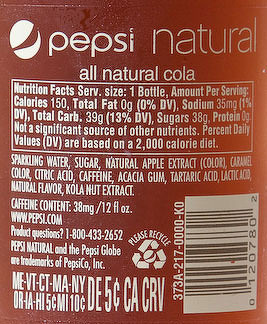The image is a close-up of the back of a bottle labeled "Pepsi Natural" with a prominent red background and white text. The label, featuring the iconic Pepsi logo partially cut off, prominently displays "All-Natural Cola" and detailed nutrition facts. Key nutritional information includes a serving size of one bottle, with 150 calories, 0 grams of total fat, 35 milligrams of sodium (1% DV), 39 grams of total carbohydrates (13% DV), 38 grams of sugars, and 0 grams of protein. The ingredients list specifies sparkling water, sugar, natural apple extract, color (caramel color), citric acid, caffeine, acacia gum, tartaric acid, lactic acid, natural flavor, and kola nut extract. Additionally, it mentions that the caffeine content is 38 mg per 12 ounces, and the website www.pepsi.com and a customer service number (1-800-433-2652) are provided. The label also includes states with deposit return information, a recycling symbol, and a barcode located in the lower right corner. Other text on the label is too small to read clearly.